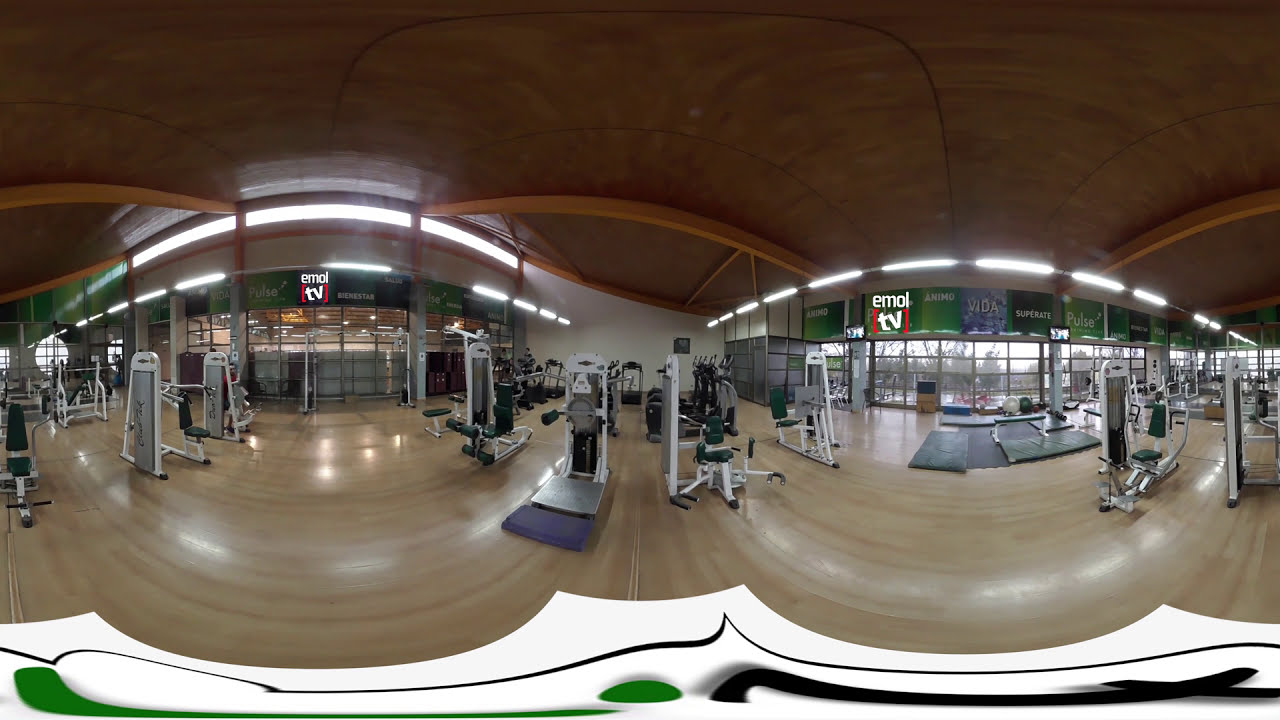The image showcases a spacious, well-lit gym with a panoramic view. The gym, possibly located in another country, features a light-colored, shiny hardwood floor reflecting the abundant natural light streaming in through numerous large windows. These windows offer a view of a bright sky and some trees outside, enhancing the airy atmosphere. Gym equipment is neatly arranged throughout the space, occupying the left, right, and center of the room. Above the windows, there's signage with multiple languages, including a prominent lit-up sign that reads "Emo TV" in red brackets and other text such as "Animo, Vita, Super," and "Pulse" on a green background. The gym appears empty of people, contributing to its relaxed and open feel. The colors present include black, silver, white, purple, blue, tan, gray, and brown, making for a visually diverse setting.